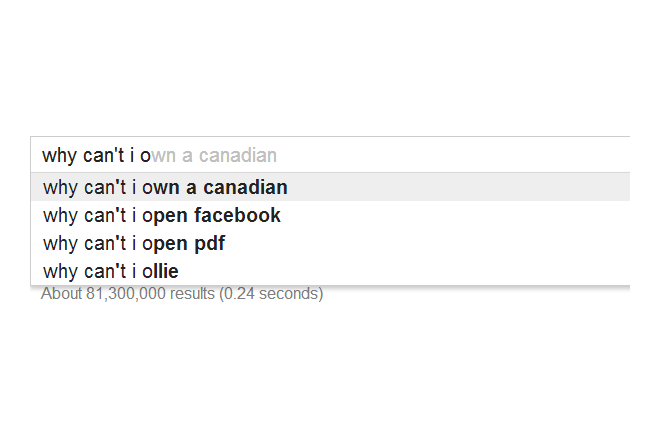This is a detailed description of the screenshot you provided:

The image is a screenshot of a search query being typed into the Google search field on a web browser. The background is white, typical of Google's minimalist design. In the search field, someone has partially typed out the phrase "why can't I O". As per Google's autocomplete feature, a drop-down menu appears with a list of suggested searches to complete the query. 

The first suggestion in the drop-down menu is "why can't I own a Canadian?" in grey text, highlighting the quirkiness of Google's autocomplete at that moment. Following this, the next suggested queries appear in a descending order: "why can't I open Facebook?", "why can't I open PDF?", and "why can't I Oli?" each reflecting common user issues or unique search attempts. 

Below these suggestions, in smaller grey text, there is a message stating "About 81,300,000 results (0.24 seconds)," indicating the number of results found and the speed of the search. The browser interface and the placement of elements all point towards it being a typical Google search engine layout.